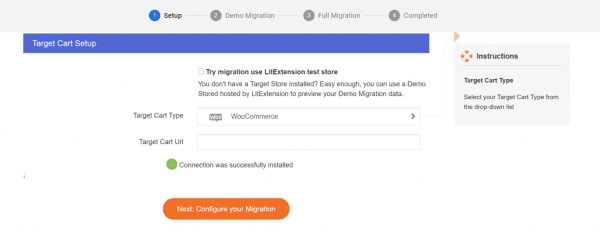The image displays a web page with a clean, white background. At the top of the page, there is a horizontal gray banner. Positioned within this banner, on the far left, is a blue circle labeled with the number "1". Adjacent to it are three gray circles, each numbered "2", "3", and "4", respectively. These are labeled as follows: "Demo Migration" for number "2", "Full Migration" for number "3", and "Completed" for number "4". 

Below this banner is a prominent blue header that reads "Target Cart Setup" in a crisp, white font. To the right of this blue header, a faded orange arrow points directionally to the right.

Beneath the header is a graphic of a life preserver, colored in white with yellow or possibly orange accents. Within the life preserver, there is instructional text stating "Target Cart Type". It elaborates further to "Select your target cart type from the drop-down list."

Centrally located on the web page is a section with the text: "Try Migration Use Life Extension Test Store. You don't have a target store installed. Easy enough, you can use a demo store hosted by Life Extension to preview your demo migration data."

At the bottom of the page, there is a large, eye-catching orange button that reads "Next Configure Your Migration".